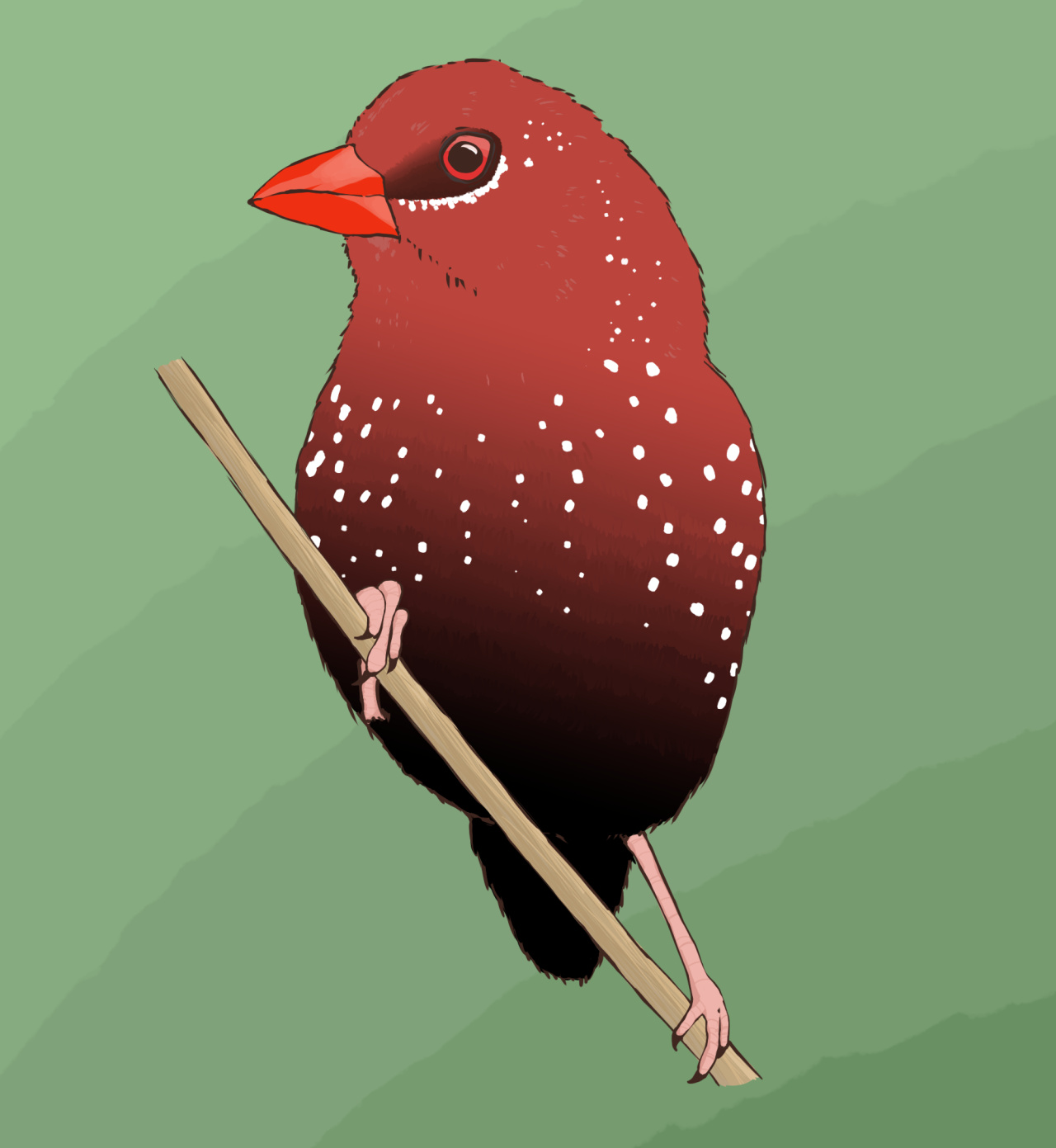This is an intricate painting of a red bird, positioned centrally in the image. The bird has a plump, maroon-colored body that gradually turns black towards its tail. The tail itself is entirely black and appears relatively fuzzy. The bird's head, with its red coloring and orange beak, is turned to the left. Surrounding the black eye, there is a red area, and a touch of white is present underneath it. White specks dot the bird’s body. The bird's talons are white and it is perched on a slender, light brown twig that extends diagonally from the bottom right to the upper left of the image. The background is comprised of varying shades of green, transitioning from lighter hues at the top left to darker ones at the bottom right, with arcs of color framing the bird.